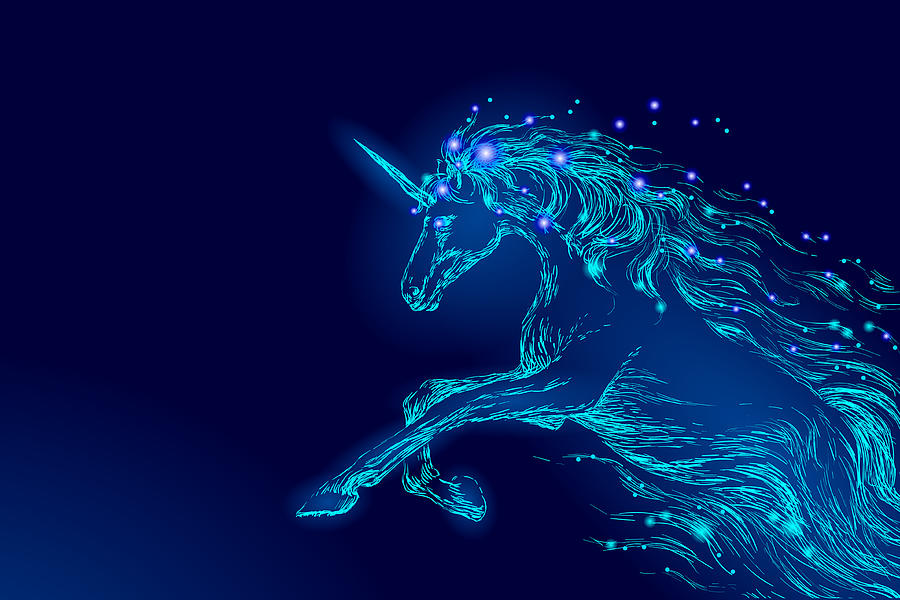The image showcases a dynamic digital graphic of a luminous unicorn, primarily positioned on the right side, against a dark blue, almost black background. The unicorn, depicted in shades of blue, appears to be leaping forward with its front hooves raised. Its distinctive long mane and sharp, glowing horn add to its majestic and mystical appearance. The creature is adorned with sparkling purple dots that glow like stars, accentuating its eyes and mane, and creating an ethereal aura around it. This artistic representation captures the essence of movement, as if the unicorn is charging forward through the night sky.